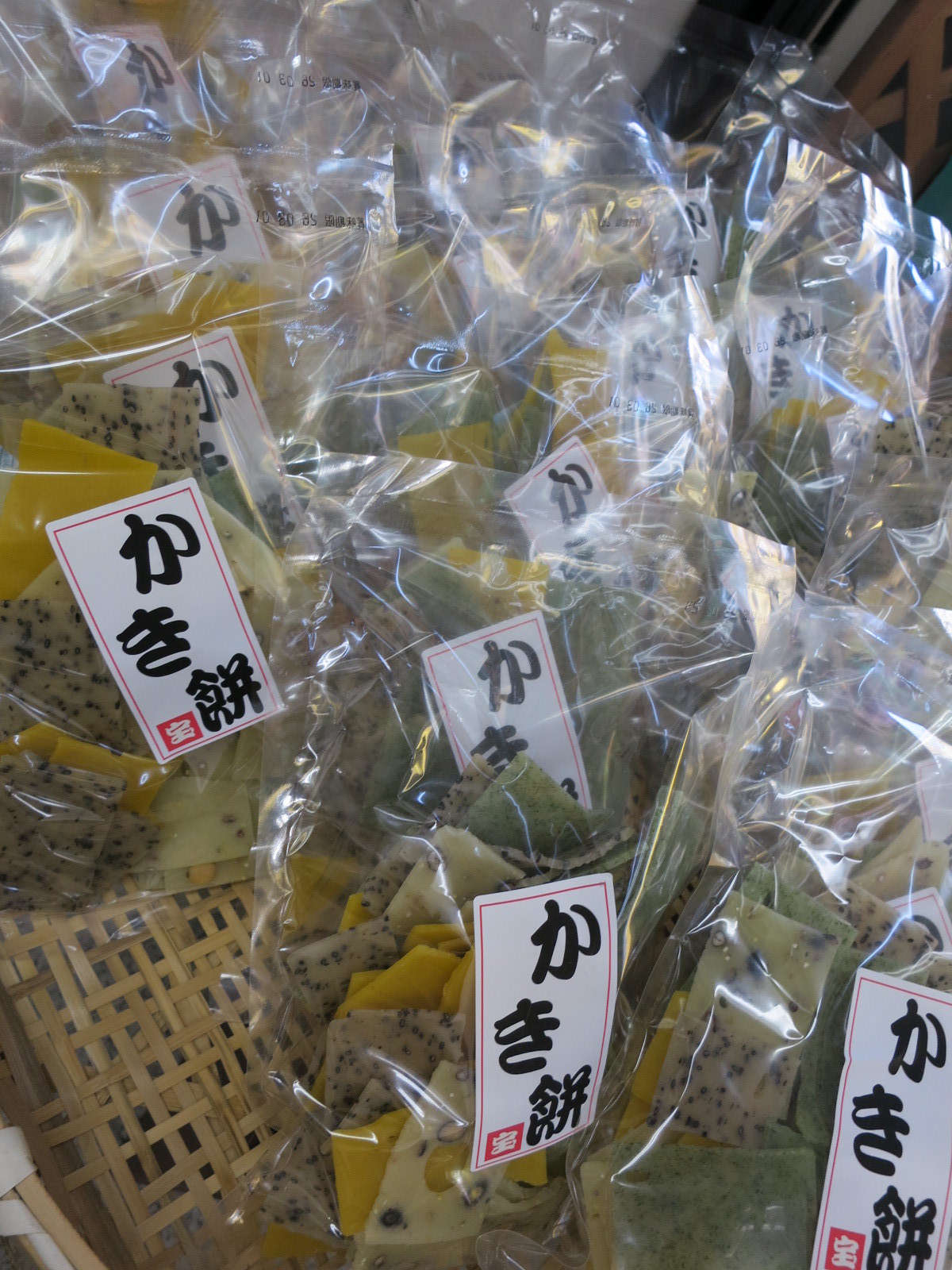The image showcases a small, light brownish-tan wooden basket with a plaid design, filled with approximately 20 individually packaged, cellophane-wrapped bags of assorted snacks. Each bag, visible through the clear cellophane, contains snacks resembling various chips or biscuits in colors such as bright yellow, white, brown, and green. The bags are neatly stacked upright and feature a white label on the front, displaying three black Chinese characters and a small red emblem in the lower-left corner. These snacks, possibly including items like sesame chips and cheese-flavored crisps, appear to be part of a gift basket arrangement.